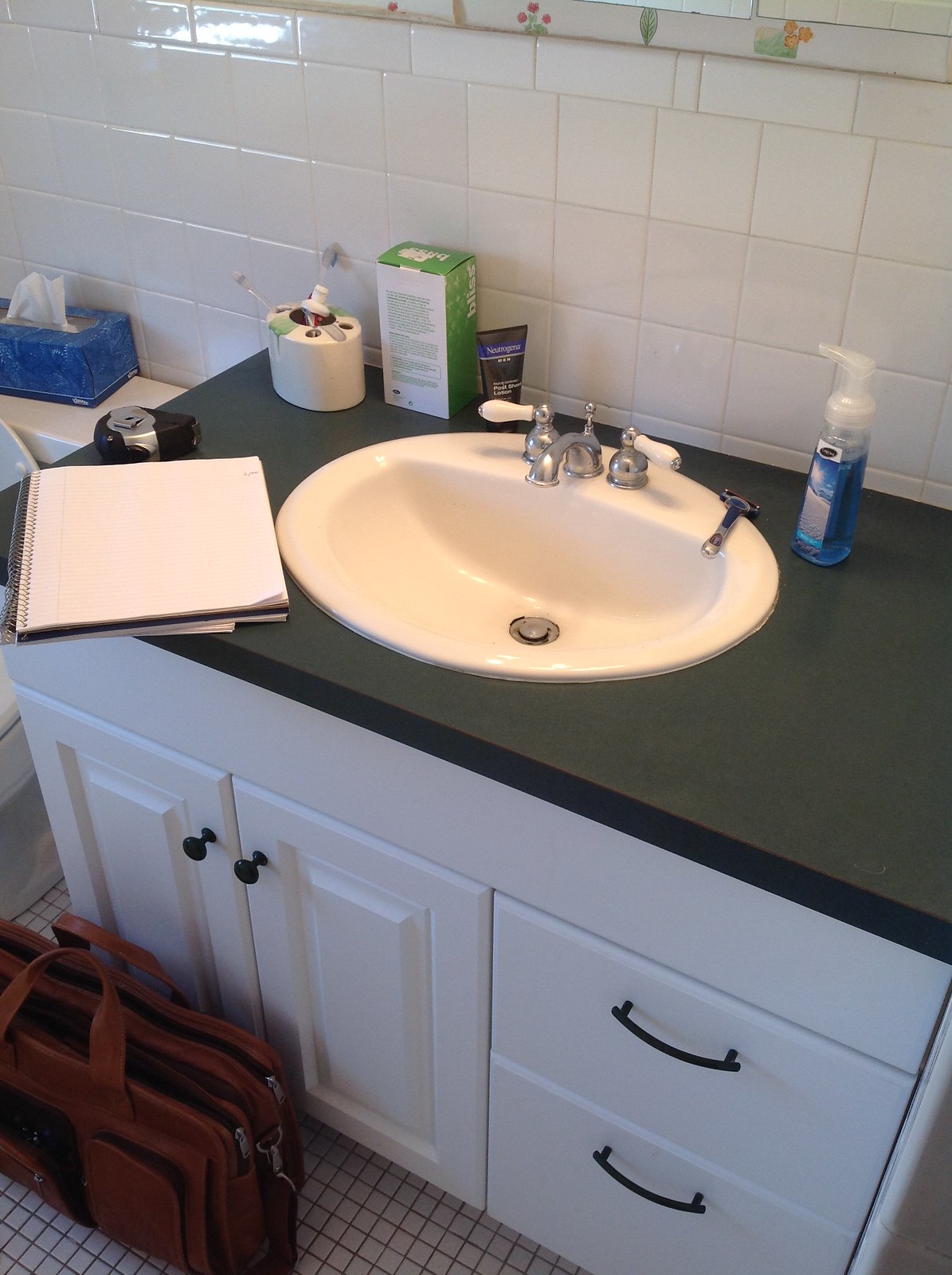The image depicts a pristine restroom setup featuring a white porcelain wash hand basin mounted on a white wooden cabinet. The basin is equipped with dull metal faucets that have white plastic handles. The cabinet itself is well-organized, consisting of two doors and two drawers for storage. On the black countertop next to the sink, an open notebook is prominently displayed. Nearby, a transparent pump bottle containing blue liquid hand-washing soap stands ready for use, along with a toothbrush holder housing several toothbrushes and two other personal care items. The floor is adorned with small, white ceramic tiles, contributing to the clean and minimalistic aesthetic. Positioned right in front of the cabinet is a stylish brown leather bag, adding a touch of sophistication to the overall setting.